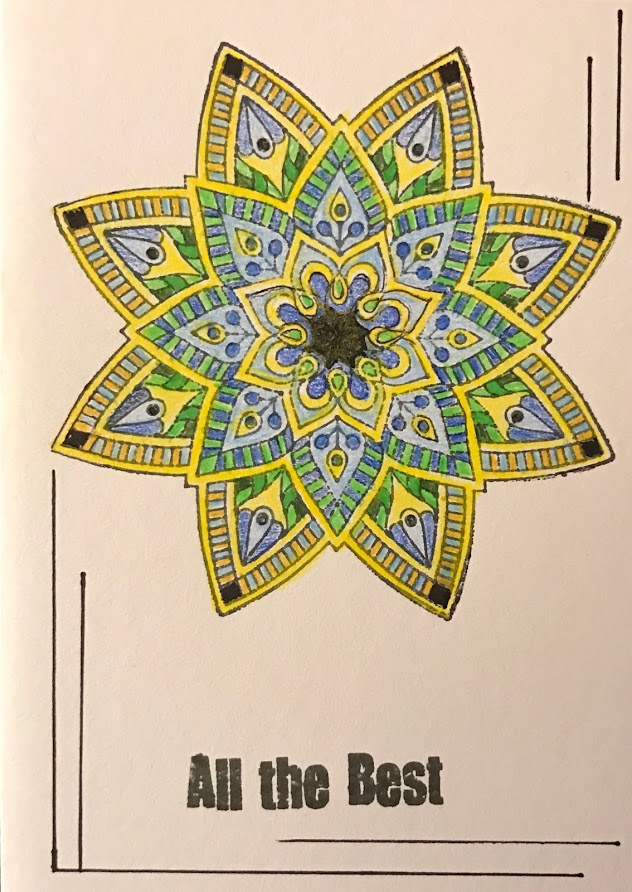This image, likely a scan or photograph of a book cover, is set against a beige background. Dominating the center is a symmetrically arranged, intricately detailed flower-like design reminiscent of an adult coloring book illustration. The flower features an eight-petaled structure that houses two smaller, overlapping floral motifs at its core. These elements radiate outwards in concentric layers, giving a sense of depth and complexity. The petals are meticulously colored with shades of blue, yellow, green, orange, light blue, and touches of black, executed with colored pencils. At the bottom of the image, in sharp black text, are the words "all the best." Additionally, the image has two black vertical poles connected by a horizontal line near the bottom left, adding to its elaborate composition.